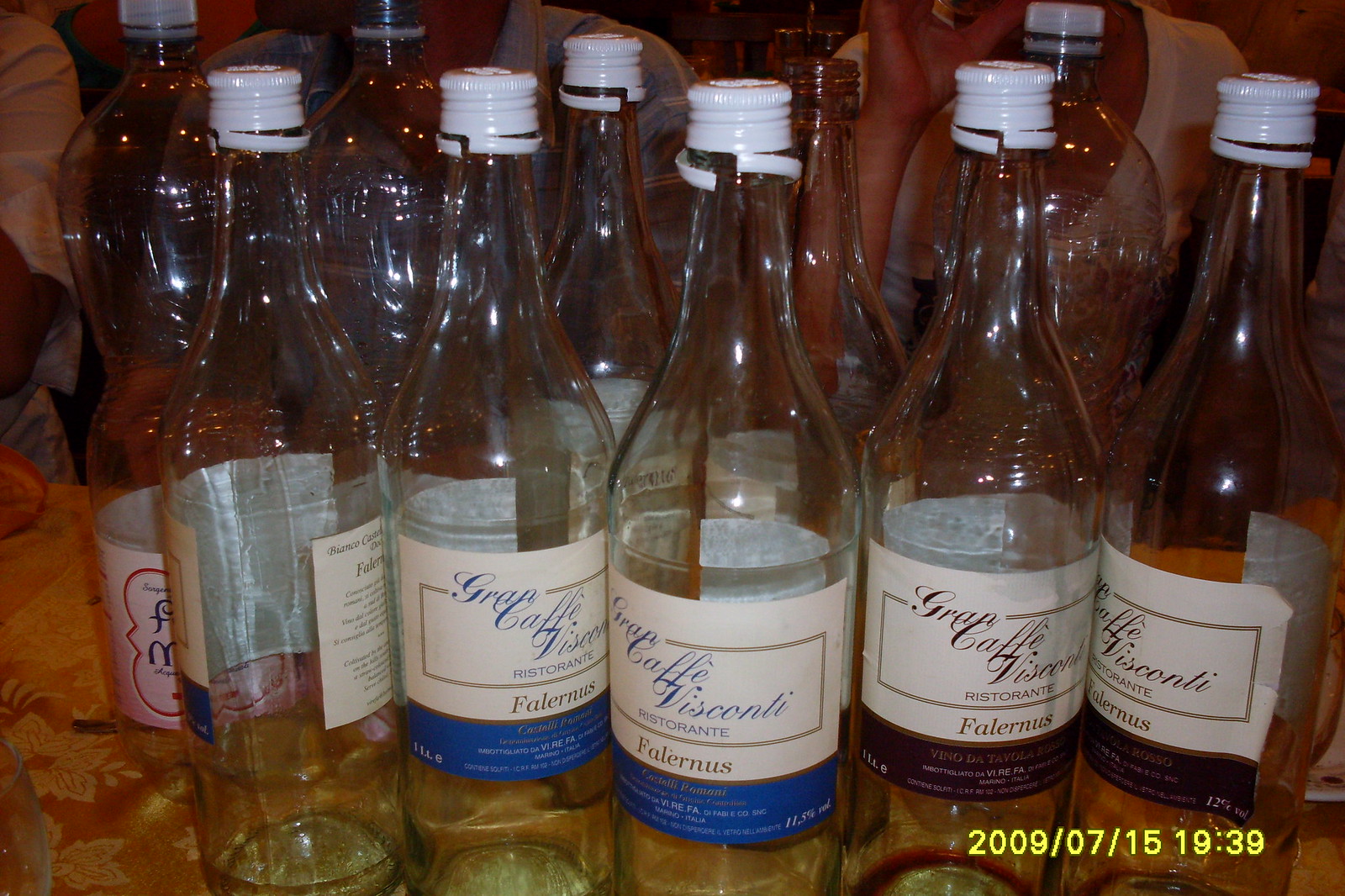The photo features approximately ten glass bottles with white metal caps, all of which are opened and mostly empty, containing only traces of liquid. The labels, written in cursive, are somewhat difficult to decipher but reveal the brand name "Caffe Visconti," suggesting it may be an Italian beverage, possibly wine. The labels display a variety of colors, including white, blue, gold, and purple. These bottles are arranged on a table covered with a tablecloth that has an orange and yellow design. In the bottom right corner, a timestamp reads "2009/07/15 19:39," indicating the image was taken digitally at that date and time. The background is nondescript, featuring at least three people blurred out, emphasizing the bottles as the primary focus of the image.